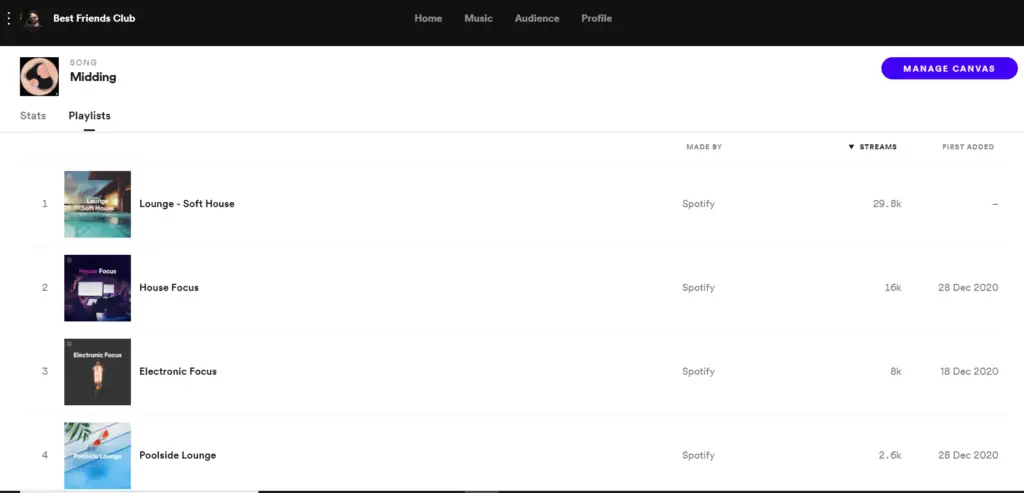**Caption:**

The image displays the "Best Friends Club" webpage, characterized by a sleek black header with white text. On the top left, the title "Best Friends Club" prominently stands out. Centrally located within the header are navigation tabs labeled "Home," "Music," and "Audience Profile." 

Positioned on the top right, just below the header, there is a blue button labeled "Manage Canvas" in white text. Just to the left of this button are additional labels including "Song" and "Meeting," accompanied by a black and brown song icon. Below these, the word "Stats" is prominently displayed.

Under the "Stats" section, there are four playlists listed, all curated by Spotify:

1. **Lounge Soft House** - 29.8k streams
   - First edit date: Not specified

2. **House Focus** - 16k streams
   - First edit date: December 28, 2020

3. **Electronic Focus** - 8k streams
   - First edit date: December 18, 2020

4. **Poolside Lounge** - 2.6k streams
   - First edit date: December 28, 2020

The entire composition is set against a clean white background, emphasizing the content presented.